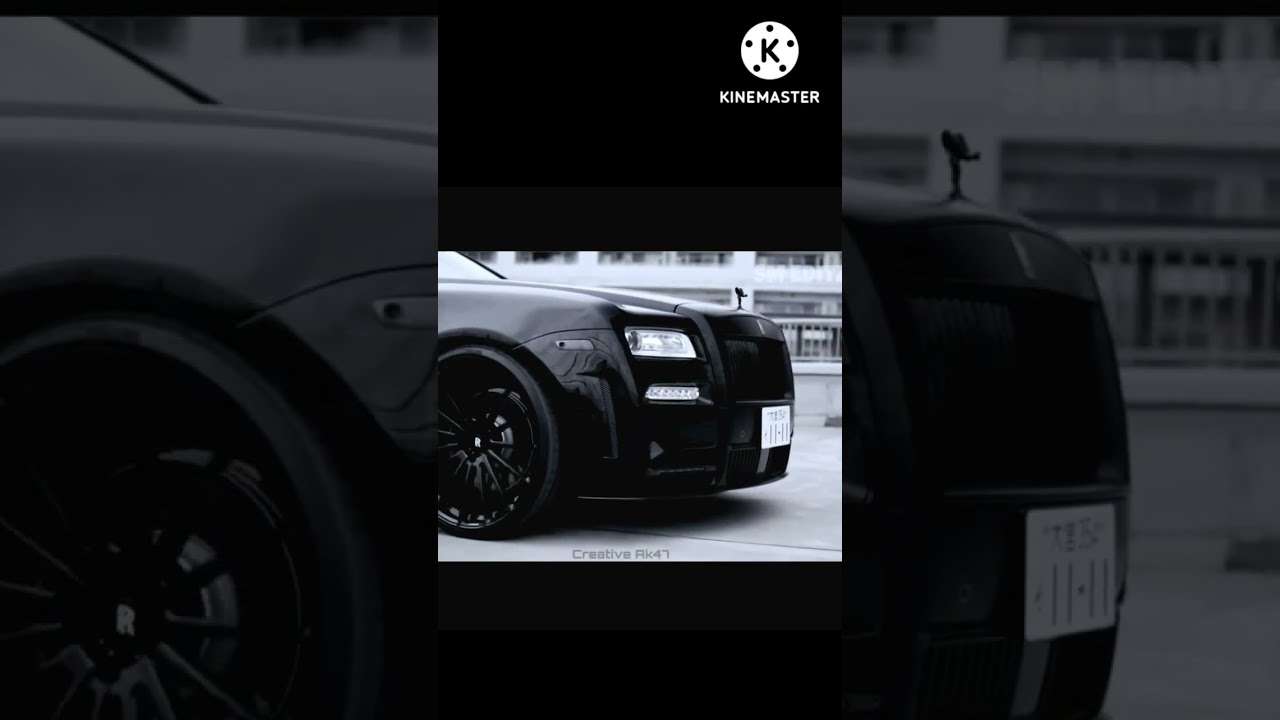This detailed depiction captures the essence of a high-end black Rolls Royce presented through a striking, tri-panel monochrome photograph. The central panel is a tall rectangle showcasing the front side of the lavish vehicle, complete with its distinct hood ornament—possibly an angel—and a white license plate. The left and right panels feature close-up, darker-shaded images of the same car, zoomed in for emphasis. In the upper right corner of the image, there is a prominent logo: a white circle with five paper hole punch-like holes around a large letter “K,” accompanied by the text "KineMaster." The entire composition exudes sophistication, accentuated by the car's black rims and shiny bright windows. Below the car image, the text "Creative AK-47" is visible, alluding to the advertisement's artistic theme. The vehicle is stationed on a street opposite a white building, reinforcing an exclusive, polished vibe suitable for such a luxury brand.